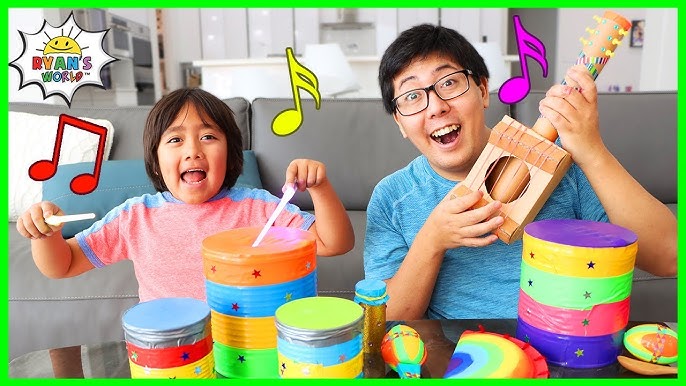The photograph is a vibrant advertisement for Ryan's World featuring a joyful scene with two figures: a young child, possibly around four or five years old, and an older male, likely the child's father or older sibling. They are both immersed in a playful and musical moment, smiling with glee. The child, seated on the left, is enthusiastically playing homemade drums with white drumsticks. The drums are vividly decorated with bright orange, blue, red, and green duct tape and adorned with shiny star stickers. The older figure, wearing glasses, is holding a makeshift ukulele or guitar crafted from what appears to be a cardboard box and a paper towel roll with plastic pins, illustrating DIY creativity. They are sitting on the floor in front of a gray-cushioned couch, with a white kitchen visible in the background. The image is framed by a fluorescent green border and includes superimposed musical notes in red, yellow, and purple, adding a whimsical touch. The top left corner features the Ryan's World logo, along with a cheerful, smiling sun icon, enhancing the playful and fun atmosphere of the scene.